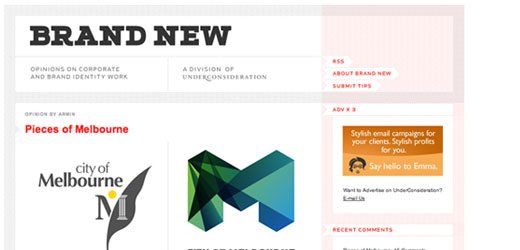In the upper left of the image, the words "Brand New" are displayed in a stylish Western-type font reminiscent of old Wild West movies. The text is in black against a white background. Beneath this, there is a description on the white background that reads "Opinions on corporate and brand identity work." To the right of this, it states "A division of Under Consideration." Adjacent to this, on a light pink background, there are three buttons labeled "RSS," "About Brand New," and "Submit Tips" with arrows that resemble flags, all featuring red lettering.

Further down, on the left side, there’s a section labeled "Opinion by." However, the author’s name is not legible. Below this, in red font, it reads "Pieces of Melbourne, City of Melbourne." The Melbourne logo depicted here is a stylized "M," where one arm of the "M" resembles a Roman column. The logo includes a yellow sun in the middle of the "M," and a feather pen's silhouette lies behind the Roman column.

To the right, there is an emerald-colored block composed of various shades of blue and green, forming another "M." Further to the right, the text reads "Stylish email campaigns for your clients, stylish profiles or products for you," followed by the phrase "Say hello to Emma." Beneath these elements, the section "Recent Comments" is located.